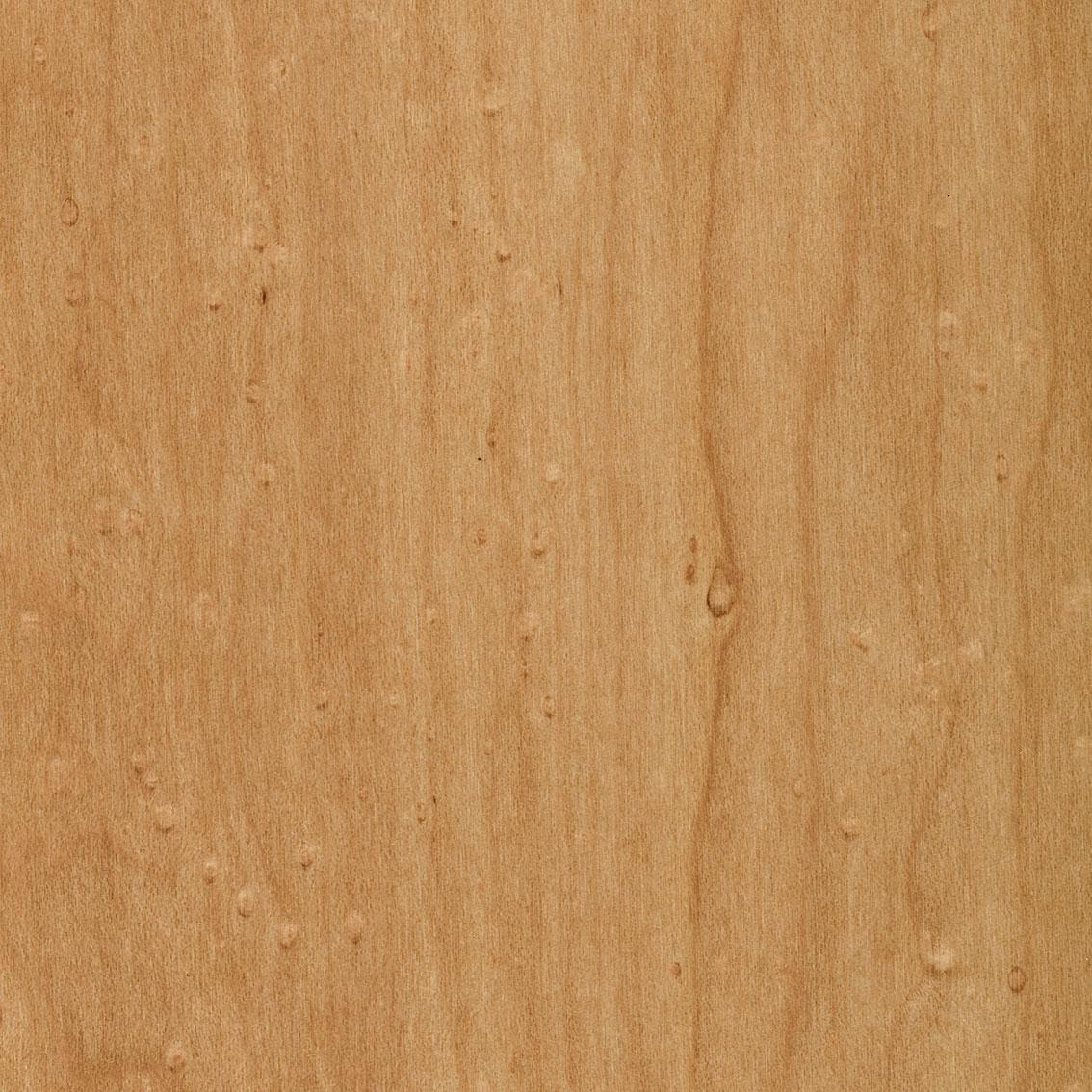The image is a detailed photograph of a light, tan, grained wood surface, possibly vinyl flooring designed to mimic natural wood. The wood appears to be a single piece without seams, featuring a pronounced grain pattern that runs vertically from the top to the bottom, approximately one-third from the right side. This prominent wavy grain is accompanied by multiple knots and irregularities of varying sizes and shapes, in shades ranging from light tan to a darker tan brown. The wood grain varies in color, starting lighter on the left side and gradually becoming darker towards the right, interspersed with water marks or stains. These details add a rich texture and complexity to the surface, making it an appealing option for home flooring. The photograph is focused solely on the wood, with no other objects, words, people, or animals in the frame, highlighting the intricate and natural beauty of the wood grain.